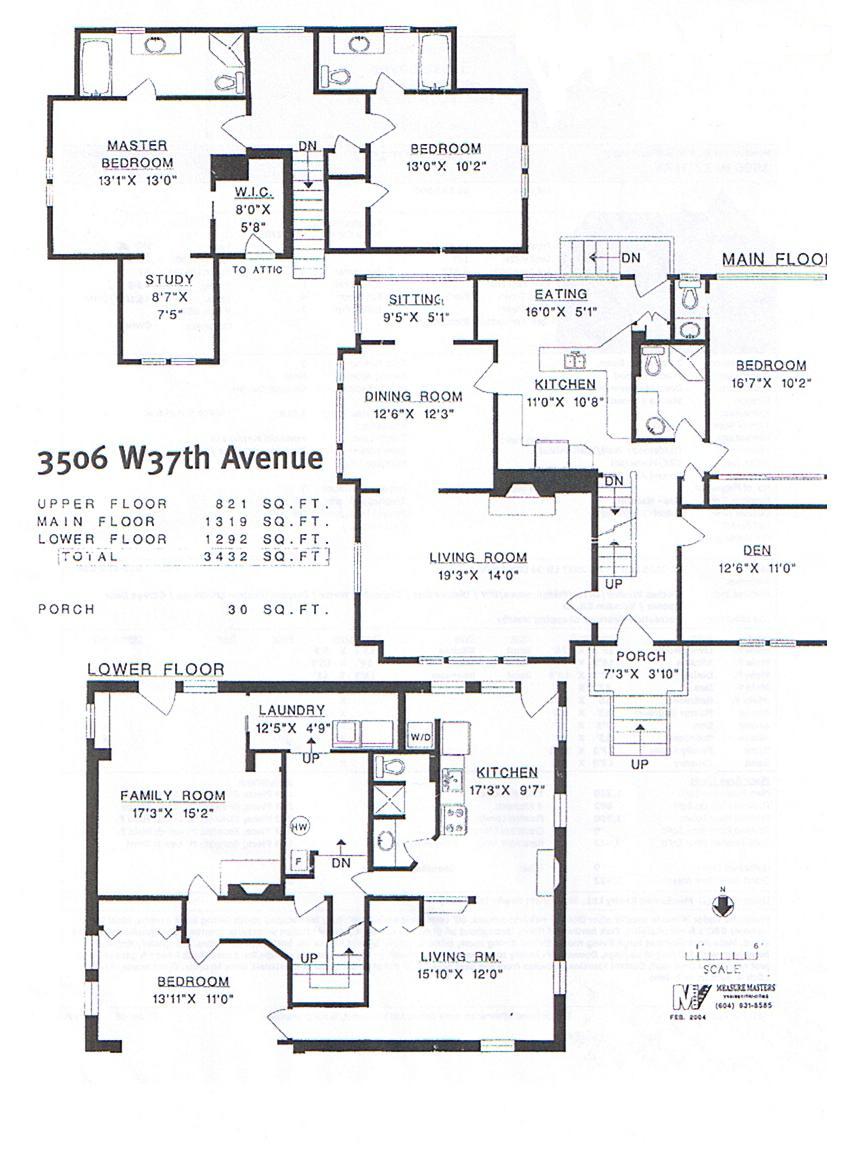### Detailed Blueprint Description of a House Design

**Location and Contact Information:**
- **Address:** 3506 W. 37th Avenue
- **Total Area:** 3,432 square feet
- **Porch Area:** 30 square feet
- **Scale:** 1 to 6
- **Design Company:** Measure Masters
- **Contact Number:** 604-831-8585

**Lower Floor (1,292 sq. ft.):**
- Designated as the "Lower Floor" at the bottom of the blueprint.
- Layout:
  - **Bedroom:** Located at the bottom left.
  - **Family Room:** Positioned at the upper left.
  - **Laundry Room:** Centrally located, connecting the bedroom and family room.
  - **Kitchen:** Situated at the upper right.
  - **Living Room:** Found at the bottom right.
- **Design Elements:**
  - Area is mostly square with a dark wood border.
  - Includes some door openings for room access.

**Main Floor (1,319 sq. ft.):**
- **Entry:** Stairs from the porch lead into a hallway.
- Layout:
  - **Den:** Located on the right side of the hallway.
  - **Living Room:** Positioned on the left, leading into:
    - **Dining Room:** Directly connected to the living room.
    - **Sitting Area:** Following the dining room.
  - **Bedroom:** Located past the den on the right side.
  - **Kitchen and Eating Area:** Situated at the front.

**Upper Floor (821 sq. ft.):**
- **Staircase Entry:** Stairs ascend to the upper floor where:
  - **Bedroom:** Located on the right.
  - **Master Bedroom:** Positioned on the left, linking to:
    - **Bathroom:** Directly connected to the master bedroom.
    - **Study:** Accessible from the master bedroom.
    - **Walk-In Closet:** Connected to the master bedroom.

This detailed blueprint provides a comprehensive layout of a multi-floor residence with precise room placements and connections, ensuring clarity for viewers or future occupants.